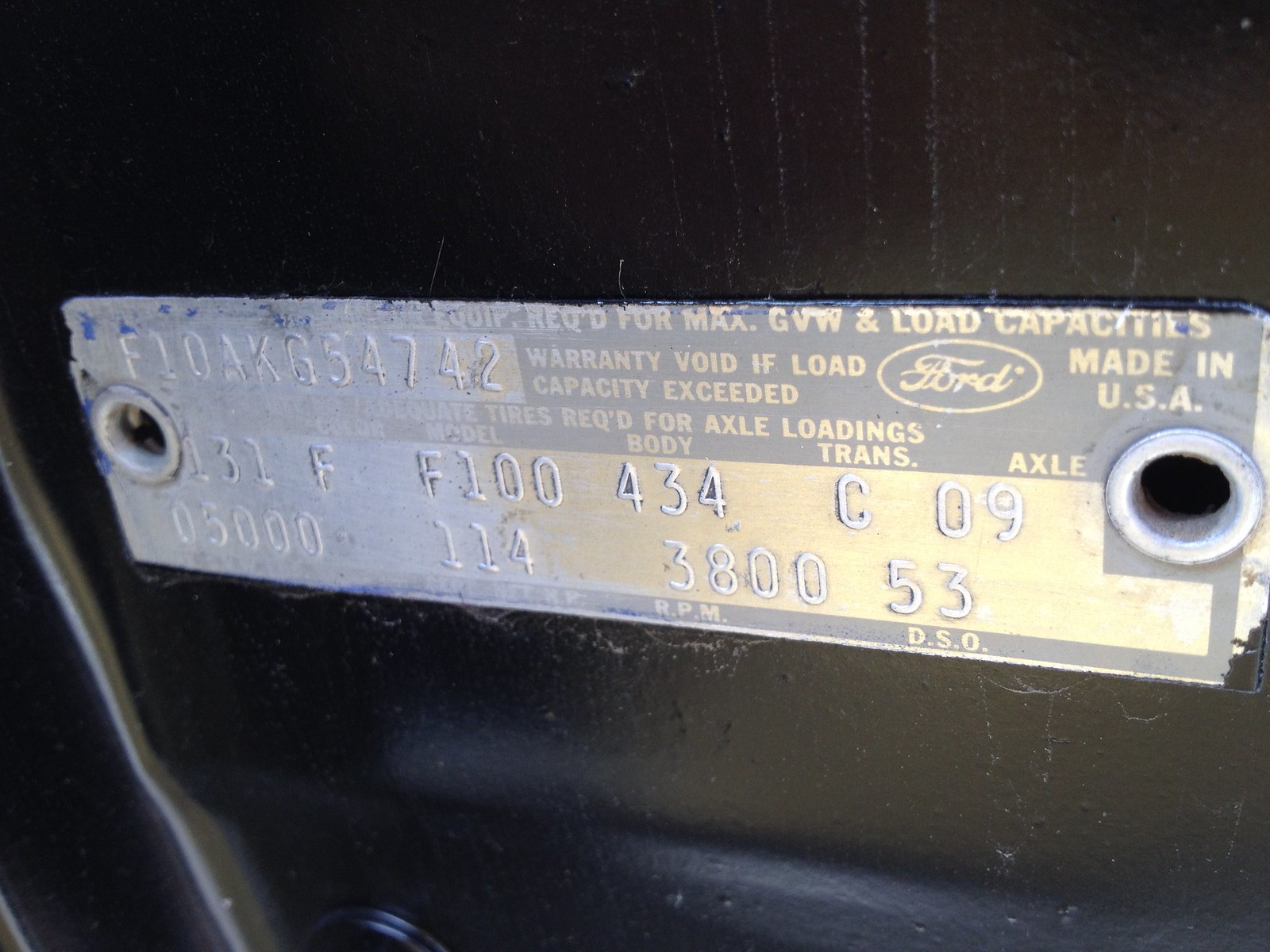The image captures a detailed view of a small rectangular metal tag affixed to the black-painted door of a Ford vehicle. The tag prominently displays several lines of information. At the top, it reads "Warranty void if load capacity exceeded," alongside the Ford logo and "Made in USA." Directly below are sections labeled "Model," "Body," "Axle," followed by a series of alphanumeric codes: "131F," "F100," "434C," and "09." Further details include numbers "0500," "114," "3800," and "53," spaced apart on the tag. This metal tag contains essential vehicle details, including load capacity and various other identification codes, crucial for understanding the specifications and warranty conditions of the car.